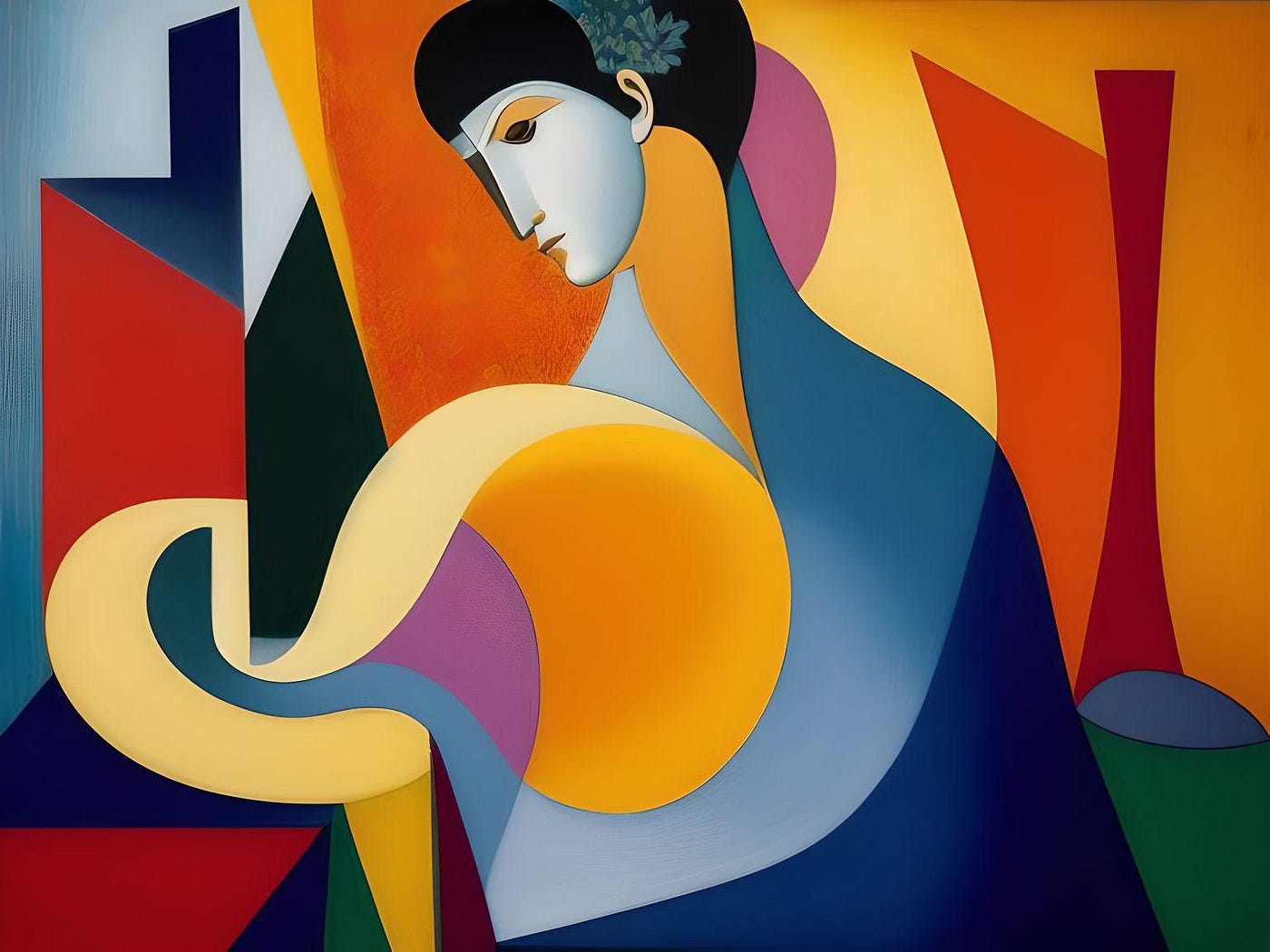This painting, with its striking abstract and Picasso-esque style, prominently features a human-like figure. The central element is a stylistically rendered face positioned towards the top and slightly oriented to the left, characterized by short black hair, a very blue elongated nose, and a mouth. The face, displaying a geisha-esque influence, includes distinctive features like a yellow ear and a combination of white and yellow tones. Below the face, the neck is depicted in yellow and transitions into abstract forms, where the blue shoulders emerge and dissolve into an array of irregular shapes. These shapes, composed of a vivid palette of colors including red, dark blue, green, purple, maroon, orange, and forest green, contribute to the modern and dynamic aesthetic of the piece. The painting’s composition lacks a background, focusing solely on the complex and colorful figure, whose simplistic shapes and lines create an intriguing and captivating visual experience.